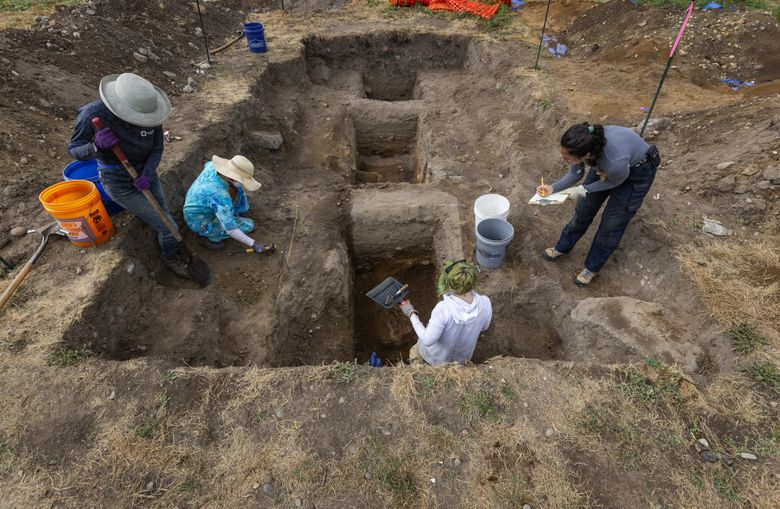This detailed image captures an archaeological excavation site where four individuals are actively engaged in digging. The scene is set within a pit that features two distinct levels, creating a ledge of dirt beneath the ground. In the upper left of the image, a person wearing a white hat is standing just inside the primary hole, holding a shovel in their right hand, with an orange bucket behind them and a blue bucket to its right. To their left, but slightly farther up in the image, another person, clad in a blue and white shirt with a yellow hat, is kneeling and seems to be meticulously scraping the dirt. In the central part of the image, several rectangular holes have been dug into the ground, each separated by a space, leading up to a T-shaped section. Inside the lower rectangle of the pit, a person in a white shirt with blonde hair is standing with their back to the camera, wielding a shovel. Above them and to the right on the ledge in the main hole, sits a gray and white bucket. Adjacent to this bucket, a person in blue jeans and a light blue shirt, with black hair, is leaning over and writing on a pad of paper. This archaeologist is positioned at the edge of the initial hole, facing left. Surrounding the pit, the ground is a mix of dirt and little patches of grass. Additional context is provided by spotting another blue pail at the upper edge of the site, hinting at the systematic and organized nature of this dig. The entire scene suggests a careful exploration, possibly of ancient remnants, with the workers equipped with shovels, brushes, and other tools to uncover and document their findings.